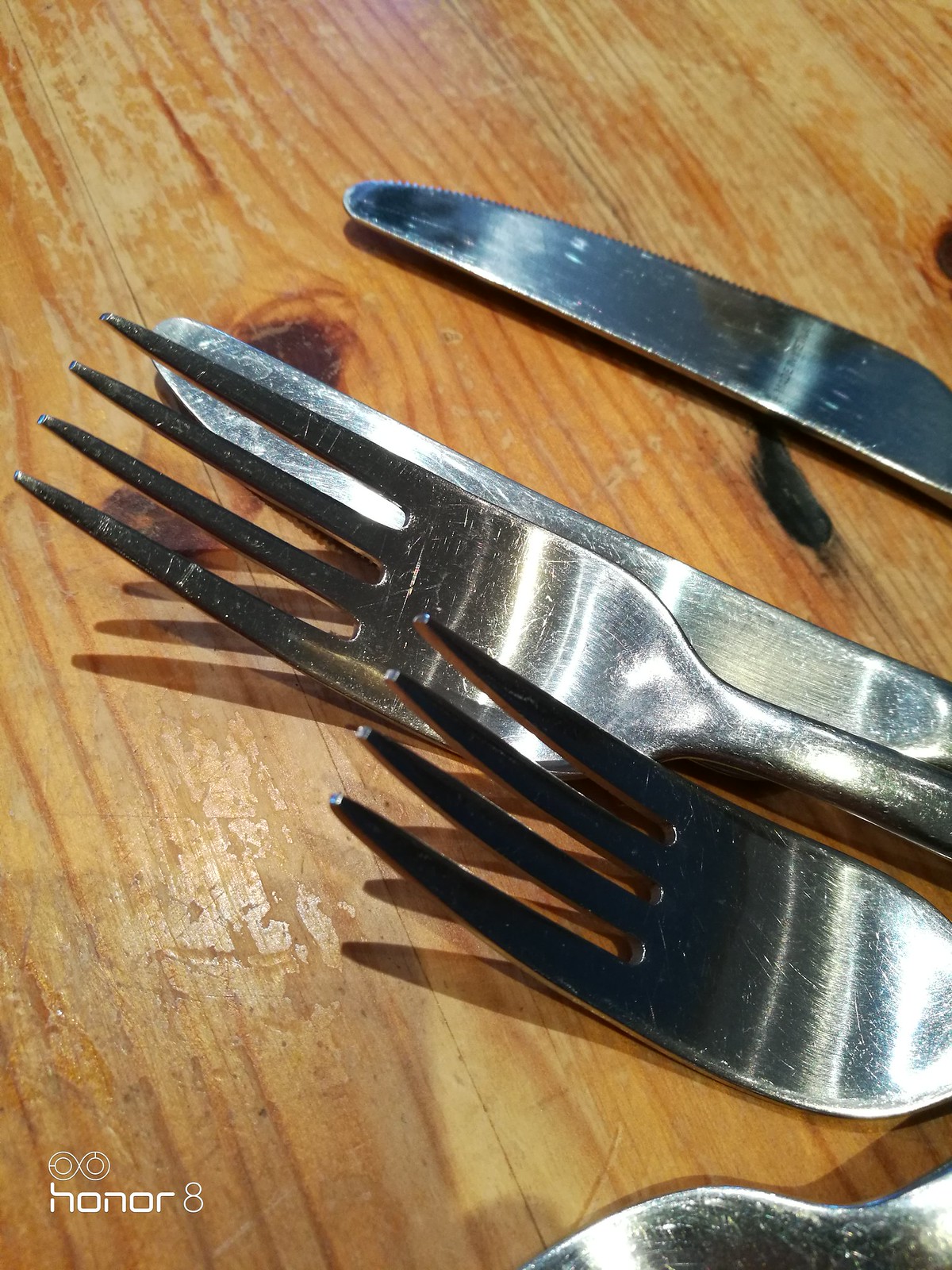The image features an arrangement of silverware on a light brown wooden table, likely made of knotty pine, displaying prominent black and brown spots and streaks in the wood grain. The table's surface looks worn, adding an aged, rustic charm. At the bottom right corner, part of a silver spoon is visible. Diagonally extending from the right side of the frame are four more pieces of silverware: two forks and two butter knives, with only their top halves in view. Notably, one fork has four prongs and resembles a dinner fork, while the other appears darker at the tips, possibly due to shadowing. In the lower left corner of the image, the text "HONOR 8" is displayed in white, accompanied by two small circles above the number 8.